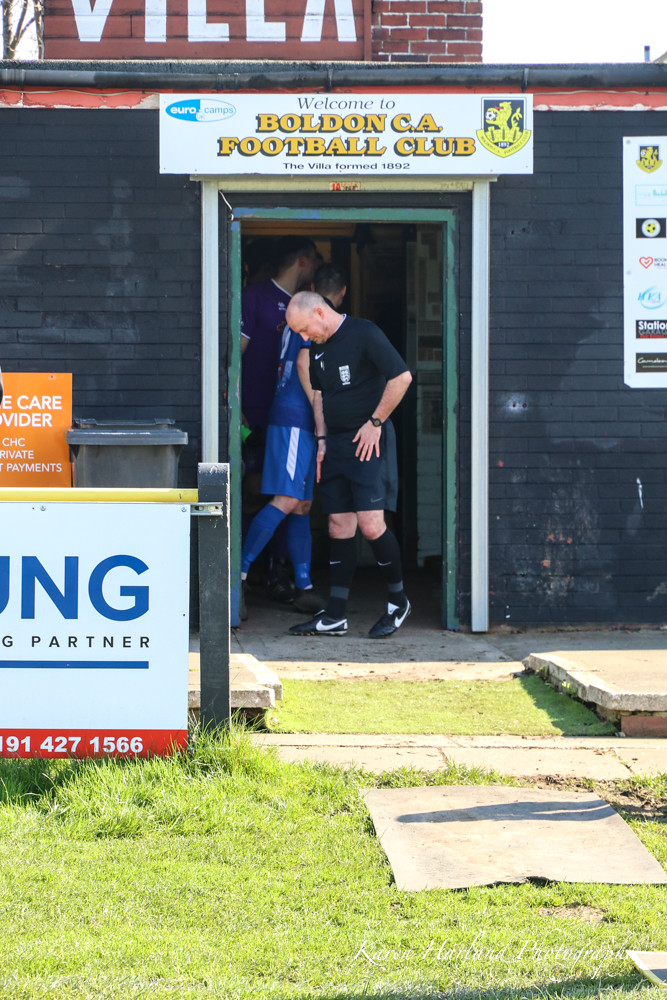In this bright, sunny outdoor image, three soccer players are seen exiting a football club building with black siding and a red chimney. The building's front door, currently open, is adorned with a prominent white sign that reads, "Euro Camps, Welcome to Baldin CA Football Club," alongside the club's crest and yellow-centered text. Partially visible on the black-painted brick structure are additional signs, including one listing sponsors and another partially obscured orange sign that mentions "care CHC payments." A concrete walkway bordered by green grass and a black mat leads up to the entrance, where a trash can is positioned beside the door. Railings nearby display another white sign with blue lettering reading "partner 914271566." The trio of soccer players, seemingly deep in conversation and not looking at the camera, is dressed in uniforms of black, blue, and purple, adding a splash of color to the scene.